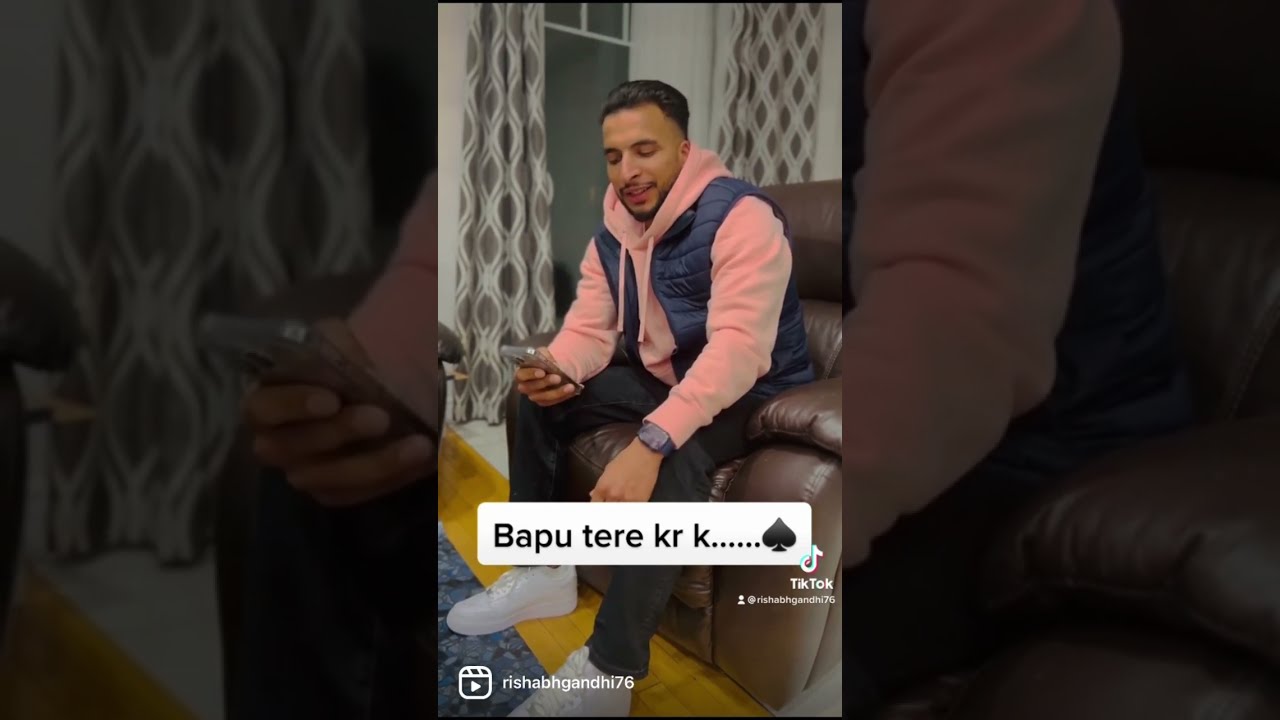The image captures a man of apparent Middle Eastern descent, seated on a brown leather armchair. He is wearing a light pink hoodie layered with a puffy blue vest, black pants, and white sneakers. A distinctive feature is his blue wristband watch. The man is engrossed in his smartphone held in his right hand and has short black hair, a mustache, and a goatee. Positioned in an indoor setting, the background reveals gray and white curtains with a window that hints at nighttime through the darkness outside. The floor's bright yellow rug is overlaid by a blue floral rug. 

The image is a screenshot from a TikTok page, evident by the TikTok watermark which includes the handle @RishabhGandhi76 on the bottom left, along with a play logo. There is additional text displayed in a foreign language, spelling out "Bapu Tere K…," followed by a black spade symbol. The same handle, Rishabh Gandhi 76, appears again, suggesting it might also be his Instagram. The screenshot features three different frames: a main shot of the man on the chair, a close-up on the left, and a zoomed-in view of his arm to the right.